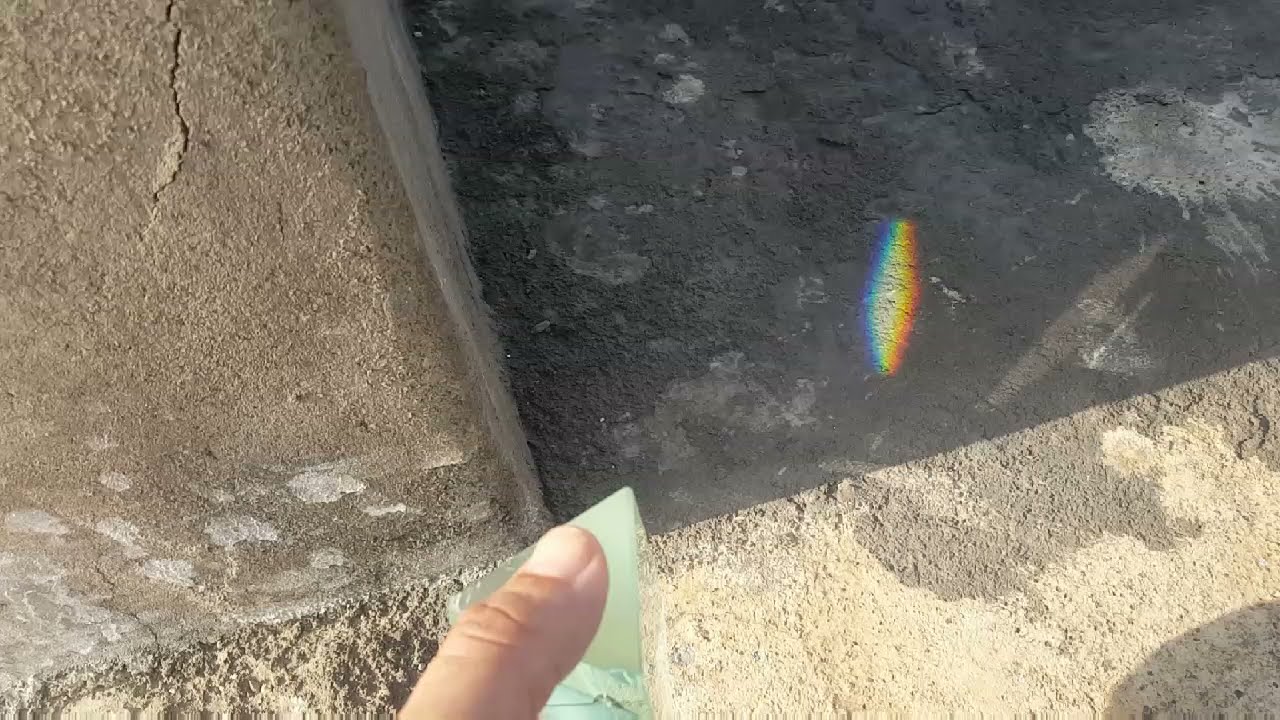In the image, a person's hand is seen holding a diamond-shaped piece of glass or mirror. The only visible part of the person is a single finger grasping the glass object. Due to the angle of the sunlight, a vibrant, prism-like reflection is cast on the floor, creating a small but striking rainbow effect. The photo is taken in the detailed corner of a room, where the walls and the floor are a matching shade of brown. The brown wall, devoid of any decoration, meets the similarly colored floor with a few noticeable white splashes scattered across it. The overall scene captures the simplistic yet captivating play of light and reflections in an understated environment.